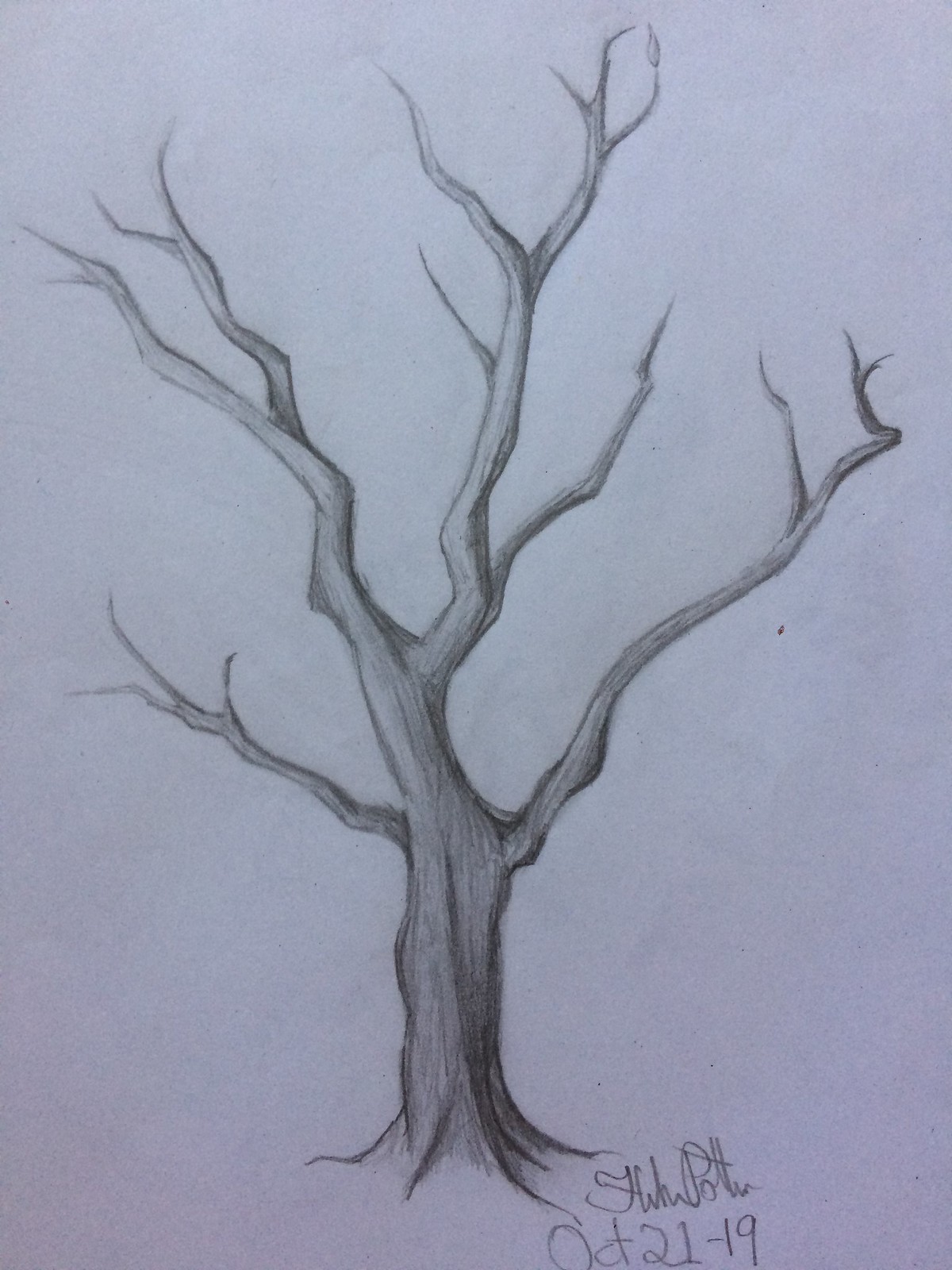Helen Potter's pencil sketch, dated October 21, 1919, features a slightly vertical composition depicting a bare tree trunk and branches. Rendered on a sketchpad, the artwork showcases intricate shading to accentuate the texture of the bark and the natural form of the branches. The trunk extends upwards towards the top of the white or off-white paper, where it splits into four main branches that fan out in opposite directions. Two additional, longer branches emerge from the lower section of the trunk. Notably, the tree is devoid of leaves or smaller twigs, focusing solely on the robust structure of the trunk and primary branches. The artist's signature and the date are positioned at the bottom right corner, adding a personal touch to this serene and detailed nature study.